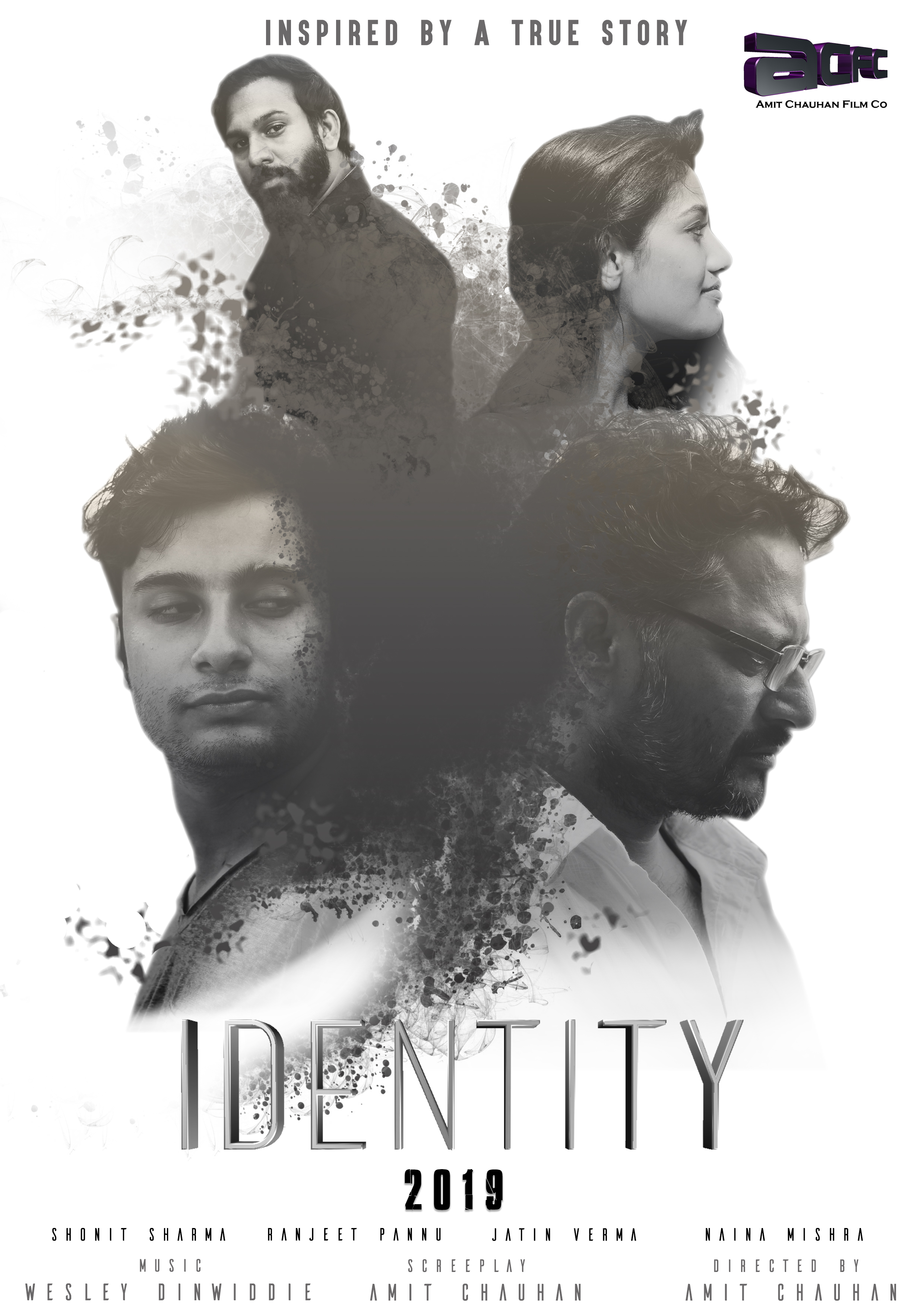The grayscale movie poster titled "Identity 2019" features four medium-skinned, dark-haired individuals arranged in a composition of two pairs. At the very top, bold black capital letters announce, "INSPIRED BY A TRUE STORY." Immediately below, the title "Identity" is boldly centered, with "2019" just beneath it. 

In the upper segment of the poster, a bearded man on the left gazes towards the viewer, while to his right, a woman smiles subtly as she faces entirely to the right. The lower section showcases two men: one on the left looks back with a pondering gaze, and the other, sporting glasses and a mustache, faces to the side with a downward, disappointed look. They contrast each other—white shirts against dark shirts, symbolizing a thematic tension. 

Names such as "Shonit Sharma, Sanjit Pang, Jatin Yerma, and Naina Mishra" appear at the bottom, alongside key credits like "Music: Wesley Dinwiddi," and "Screenplay & Direction: Amit Chiran," giving a clear preview of the film's creative crew.